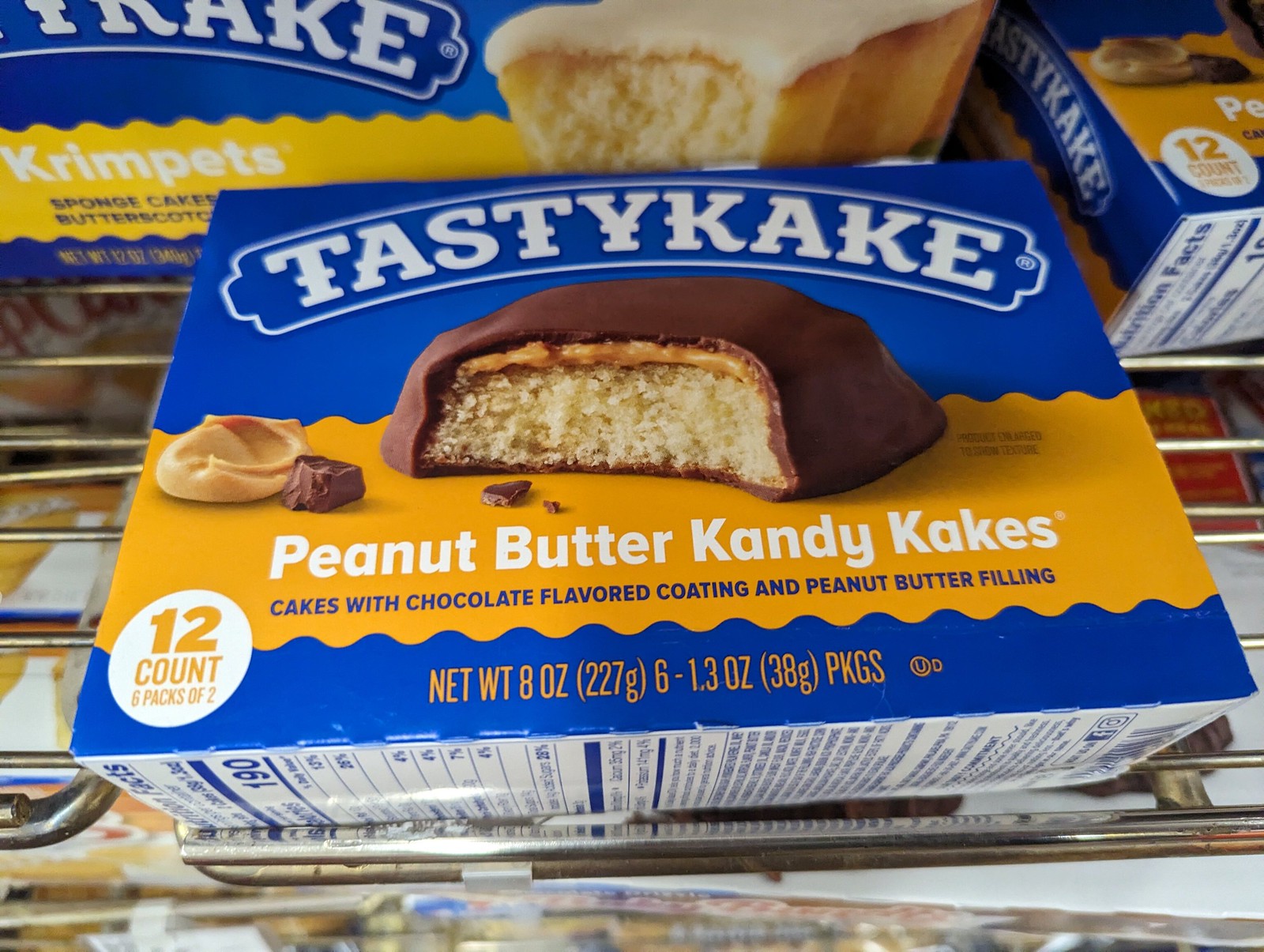The image is a top-down view of a grocery store shelf displaying a box of Tasty Cake’s peanut butter candy cakes. The metal wire shelf, made up of several long rods, has visible gaps. The focal point is the blue packaging of the Tasty Cake box, adorned with white text and a white curved border around the brand name. The main image on the box features a peanut butter candy cake covered in chocolate with a large bite taken out, revealing a vanilla-like cake with a peanut butter filling. Notable design elements include a wavy orange segment at the bottom, indicating "12 count, 6 packs of 2, net weight 8 ounces (227 grams), 6 (1.3 ounce) packages." There are also images of a peanut butter swirl and a chunk of chocolate. Additionally, a background box of Tasty Cake’s crimpets—sponge cakes with butterscotch flavor—is partially visible, along with another peanut butter candy cake box on the right. The box also indicates "190 calories" and describes the cakes as having a chocolate-flavored coating and peanut butter filling.